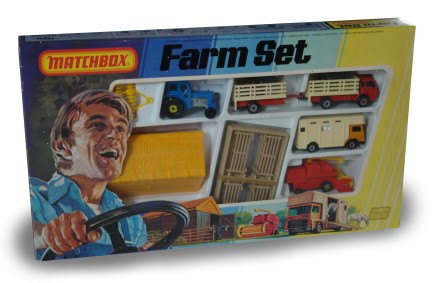This product listing image showcases a vintage 1970s Matchbox Farm Set, staged on a white surface with a white background, creating the illusion of floating in a featureless void to focus attention solely on the product. The set is encased in its original packaging, a vibrant box designed with blue, yellow, and gray tones, featuring a prominent drawing of a smiling man, presumably driving a tractor, rendered in a 1970s illustration style that might be oil paint. The Matchbox logo adorns the top left corner of the package in red text on a yellow rectangular background, above black text that reads "Farm Set." A clear plastic window reveals the toys inside: a red pickup truck with a trailer, a blue tractor, an RV, a combine, and an animal pen, evoking a sense of nostalgic charm for classic farm-themed playsets.